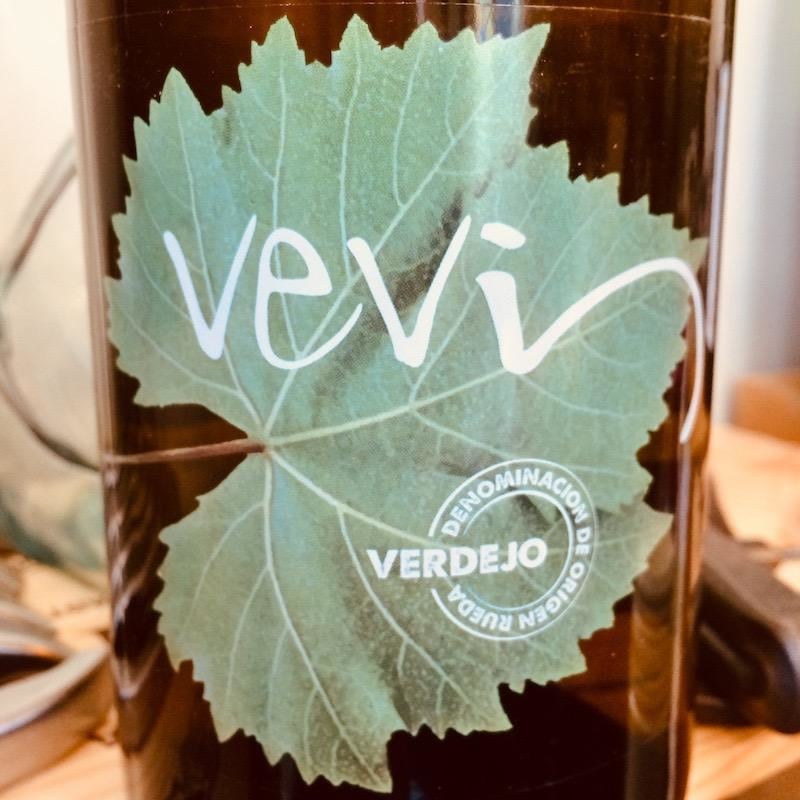This close-up photograph features a light green leaf attached to a cylindrical container, possibly a glass or pitcher, filled with a golden-brown liquid. The leaf prominently displays the white text "VEVI" and a circular white logo with the words "Denominación de Origen Rueda" encompassing the top and bottom parts, and the word "VERDEJO" cutting through the center. The container is placed on a light wood table, while the background remains indistinct and blurred, adding to the ambiguity of the setting. On the right side of the frame, a vague shape, possibly a bag, can be seen, and on the left, some unidentifiable objects rest on the table, with a blurry wall behind them.